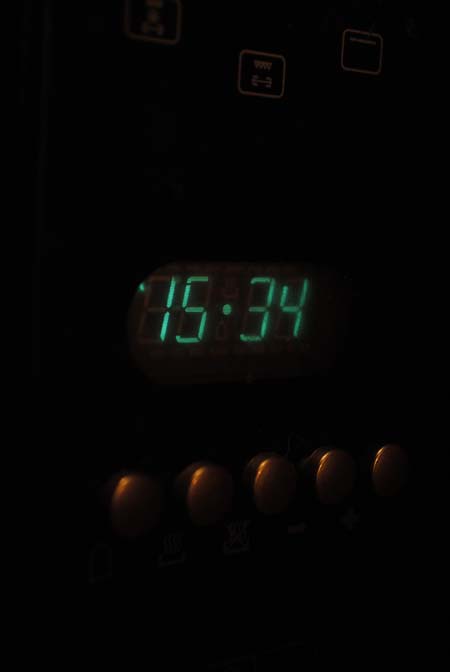The image depicts the front panel of an unidentified electrical device set against a completely black background. Dominating the center of the image is a green LED digital clock displaying the time "15.34." The green seven-segment display is bright and clearly visible. Below the digital clock readout, there are five small, dimly lit, orange lights that seem to be part of the device, possibly indicating controls or buttons. The rest of the device is shrouded in darkness, making it difficult to discern any additional features or the device's purpose, which could range from a video recorder to a hi-fi system. However, the focus remains on the digital clock and the faint, orange-lit indicators below it.